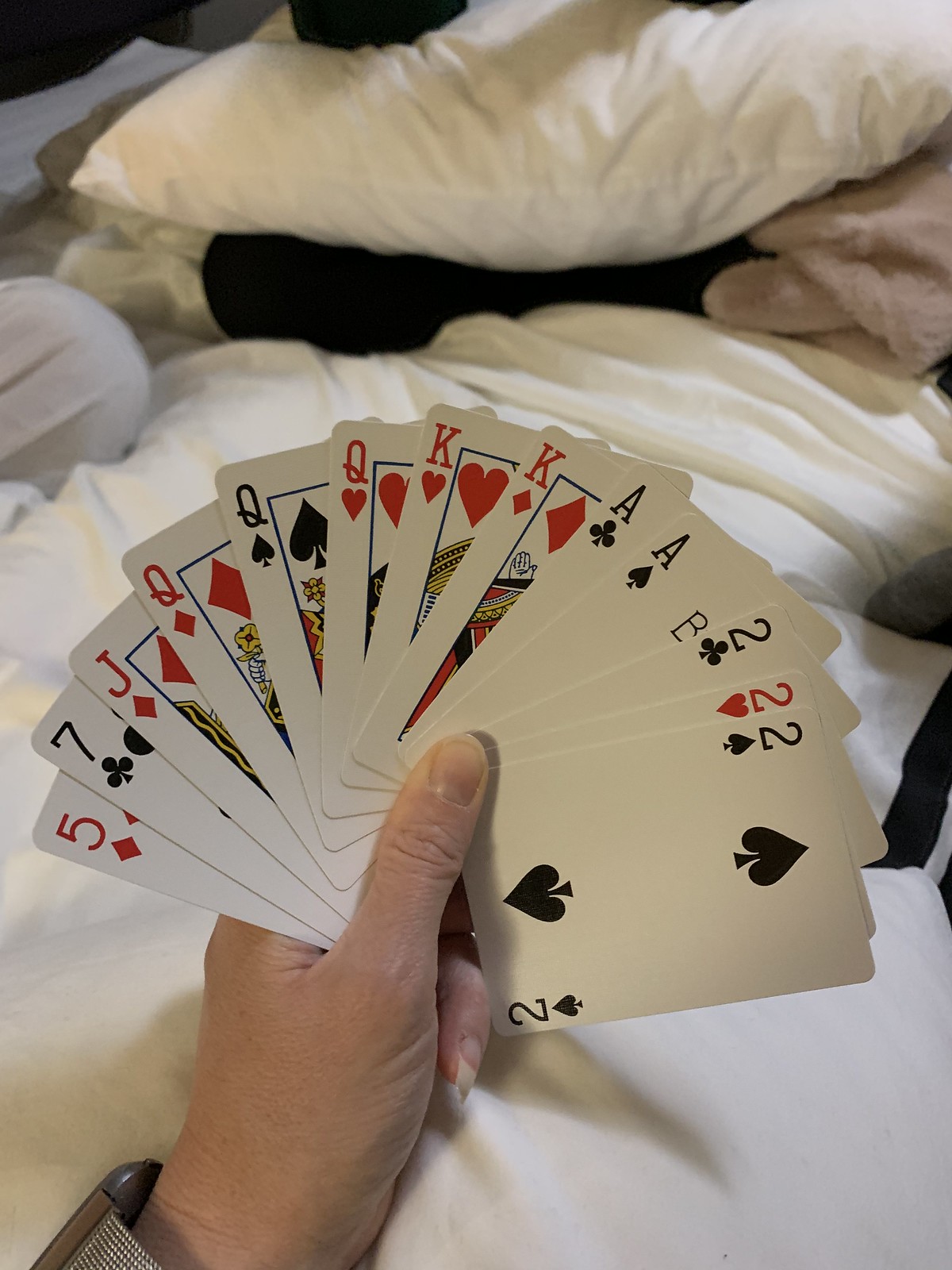The image depicts a person holding a fanned-out arrangement of playing cards in their left hand. The cards, spread from left to right, include: Five of Diamonds, Seven of Clubs, Seven of Diamonds, Queen of Diamonds, Queen of Hearts, Queen of Hearts, Queen of Spades, Queen of Hearts, King of Hearts, King of Diamonds, Ace of Clubs, Ace of Spades, Two of Clubs, Two of Diamonds, and Two of Spades. A wristwatch is visible on the person's left wrist, hinting at the time. In the background, there is a white cloth and a white pillow, suggesting the setting might be a bed. It looks like someone is resting on this bed, adding a casual, relaxed atmosphere to the scene.